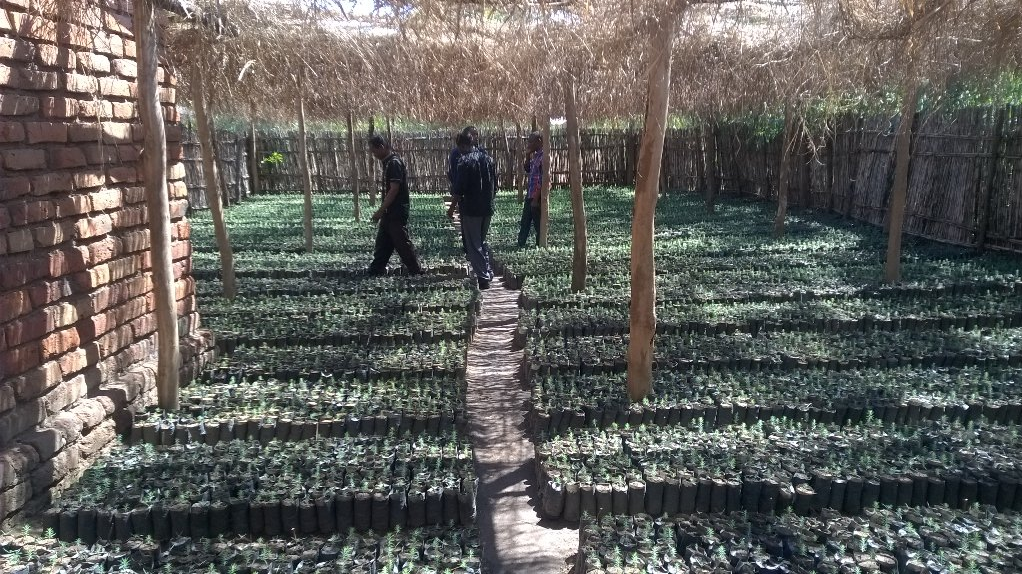The image depicts a sunny day at a gardening nursery or an area dedicated to growing various plants. On the left side of the image, there is a red brick building surrounded by wooden fencing, which encloses the entire area. The ground is covered with numerous small plants, some of which are organized in little black containers, possibly ceramic pots. There is a narrow walkway that winds through the field of plants. Overhead, a pergola made of netting with dried brown branches and leaves provides a partial covering. In the background, four individuals dressed in black are seen walking along the walkway, appearing to be in conversation and looking down at the plants. The overall color palette of the scene includes shades of green from the plants, tan, darker brown from the wooden structures and dried branches, red from the brick building, and black from the individuals' outfits. The sun shines through the pergola, casting light and shadows across the scene, adding to its vividness.